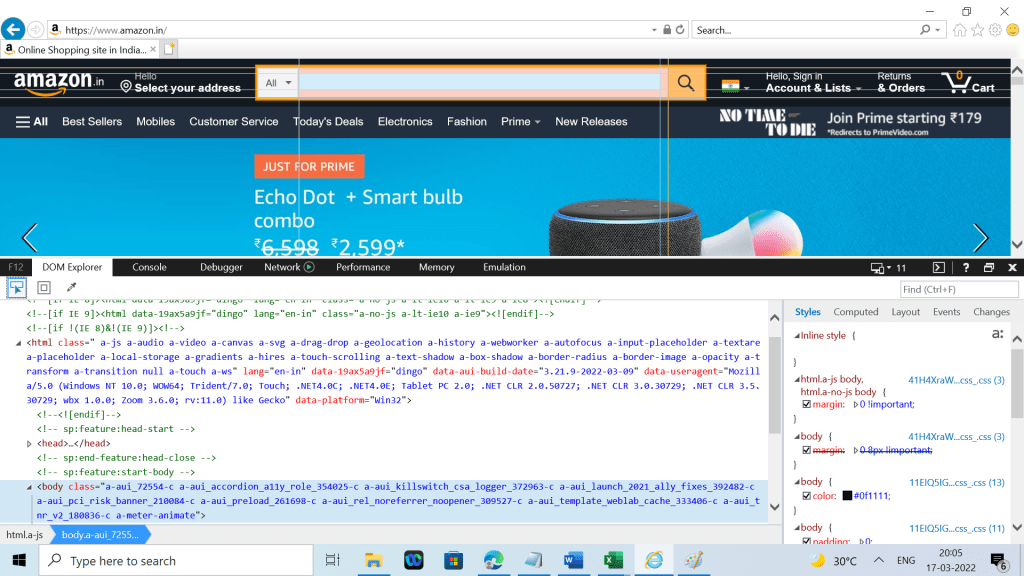Screenshot of an Amazon India Web Page with Developer Tools Open

This image is a detailed screenshot of a browser displaying the Amazon.in web page for India, as indicated by the URL and the tab title, "Online Shopping Site in India." The top section of the browser shows the main header which includes various functional tools: a search bar, options to select your address, sign in, view your cart, and access return and order information.

Below the header, there are several tabs for navigating different product categories such as Best Sellers, Mobiles, Customer Service, Today's Deals, Electronics, Fashion, Prime, and New Releases. The primary banner prominently features a promotional offer for a Prime-exclusive deal on an Echo Dot and Smart Bulb combo.

The unique aspect of this screenshot is that the browser's Developer Tools are open, specifically showing the "DOM Explorer" tab. The developer is examining the website’s underlying HTML and CSS code, with highlighted sections in blue and orange corresponding to elements likely related to the search bar. 

At the bottom of the screen, the Windows taskbar is visible, showing the user's currently active applications, including Excel, Notepad, Word, Internet Explorer, Paint, and File Explorer, along with the Windows icon and a search bar.